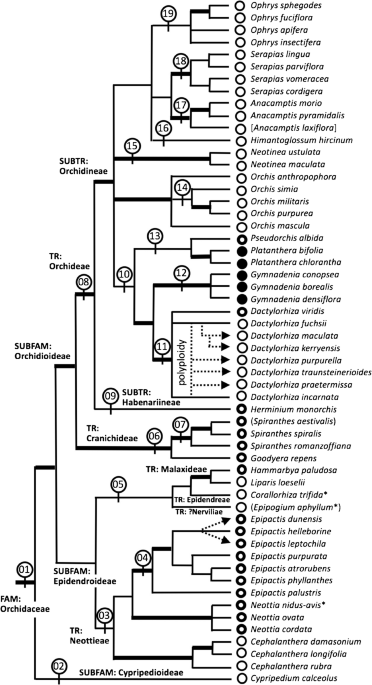The image is a highly detailed digital creation composed entirely of Latin words, with no English translations. On the right-hand side, there is a long list of double-barreled Latin words, each accompanied by a unique symbol to its left. These symbols vary: some are simple circles, others are thick black doughnut-like circles, and some are completely filled-in black circles. All these elements are left-aligned for neat organization.

Interconnecting these circles is a series of intricate interlocking lines, resembling a family tree or an elaborate category chart, with a structure somewhat akin to an NCAA tournament bracket. This tree-like diagram appears to map out a hierarchical or categorical relationship among the words. To the left of the various circles, numbers within smaller circles branch off from the horizontal lines, indicating subcategories within larger groups.

The lines connecting these elements also vary; some look like forks with two prongs while others have more substantial branches. Additional labels, also in Latin, appear along some of these horizontal lines, further detailing the relationships within the diagram. These elements collectively form a complex and thorough visual representation, likely indicating an extensive taxonomic or categorical structure.